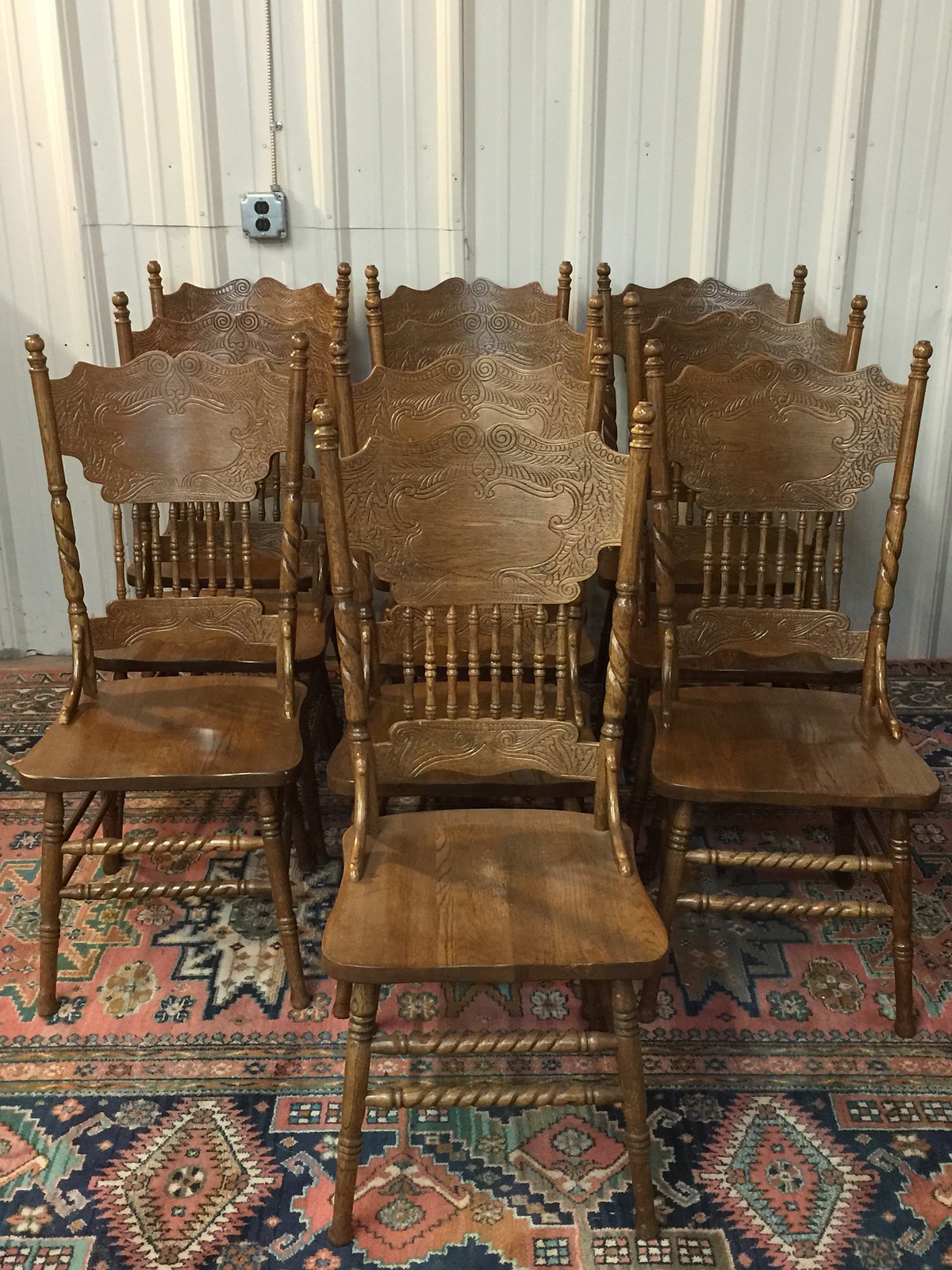The photograph features an ornate oriental carpet that exhibits a somewhat aged and worn appearance. The carpet, resplendent in hues of red, black, tan, cream, and orange, is adorned with intricate diamond and cube shapes, and detailed patterns. Atop this carpet, arranged in three rows with three across, sit ten identical wooden chairs reminiscent of 1940s dining room chairs. These chairs, crafted from dark brown or dark maple wood, feature moderately ornate carvings on the legs and side pieces that support the back. The arrangement of the chairs is symmetrical, except for the central front row, which has an additional chair positioned slightly closer to the camera. The setting appears to be a warehouse or industrial space, as indicated by the textured metallic white wall in the background, complete with a visible silver outlet on the upper left side of the image.